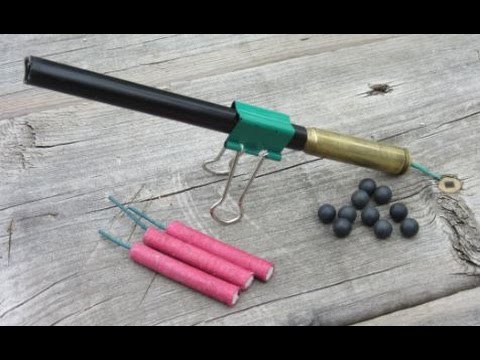This detailed photograph captures the setup of what appears to be a homemade fireworks launcher or cannon, meticulously arranged on a weathered outdoor picnic table. Dominating the mid-ground is a black, sawed-off tube with a gold base, propped up by an upside-down, teal green binder clip, giving it a makeshift yet functional appearance. To the left foreground, three red firecrackers with blue fuses are neatly placed, while the right foreground features around a dozen small black balls, reminiscent of cherry bombs or even blueberries, acting as propellant. The scene exudes a DIY Fourth of July vibe, hinting at a child's anticipation for a festive firework display.